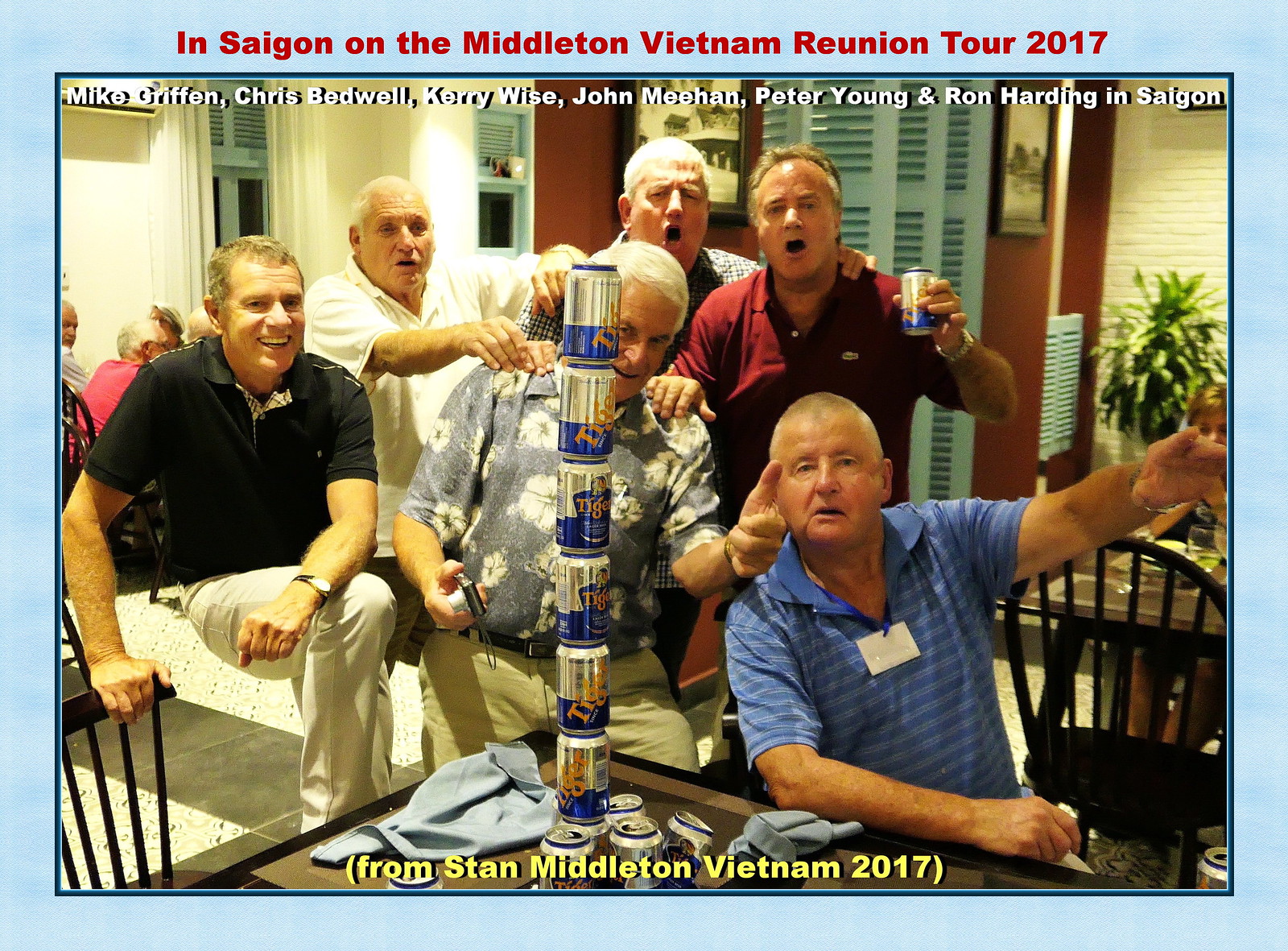This photograph, taken indoors, captures a lively scene featuring six elderly men identified as Mike Griffin, Chris Bedwell, Carrie Wise, John Meehan, Peter Young, and Ron Harding, all in Saigon. These men, seemingly in the midst of celebration, are gathered around a rectangular gray and black table, either sitting or standing. One man is seated with his hand resting on the table while the remaining five are standing. Central to the table is a striking tower of beer cans, stacked seven high, featuring the brand "Tiger" in blue, silver, and yellow colors. Additional beer cans and light blue cloth napkins are scattered across the table.

Around the photo is a light blue border. At the top, written in red text, is "In Saigon on the Middleton Vietnam Reunion Tour 2017." Just below this in white text are the names of the men from left to right: Mike Griffin, Chris Bedwell, Carrie Wise, John Meehan, Peter Young, and Ron Harding. The bottom of the picture is inscribed with "From Stan Middleton Vietnam 2017" in yellow text. The scene appears to be set inside a restaurant, as suggested by the background featuring light blue doors with vents, a burgundy or brownish-orange wall, and framed black-and-white photographs. The men are dressed in collared shirts and slacks of various colors, and a few of them are cheerfully holding up beer cans, adding to the festive atmosphere.